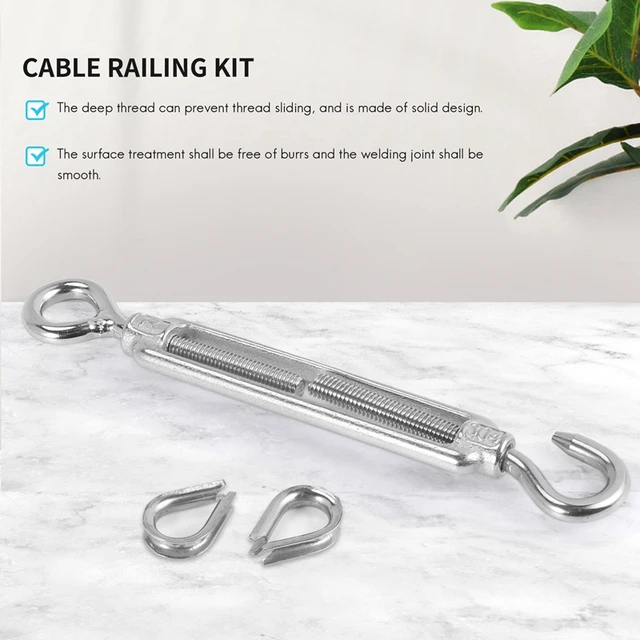This advertisement for a cable railing kit showcases the product against a pristine white backdrop, featuring a white wall and a white marble tabletop. In the left corner, a touch of greenery with four leaves adds a hint of nature to the otherwise minimalist setting. Dominating the top right of the image, bold black block letters spell out "Cable Railing Kit," accompanied by two blue check boxes. The first check box highlights that the "deep thread can prevent thread sliding and is made of solid design," while the second box assures that "the surface treatment shall be free of burrs and the welding point shall be smooth."

Central in the image is the cable railing kit itself, a sleek, long silver piece of hardware. The kit comprises two sections: the back section is circular and slopes downward from right to left, ending in a hook. Additionally, there are two more hooks laid neatly on the table in front of it. The metal piece has a loop on one end and threaded components, suggesting its adjustable nature for lengthening or shortening. This clean, modern piece of equipment is notably polished and free of imperfections, emphasizing its robust and precise craftsmanship.